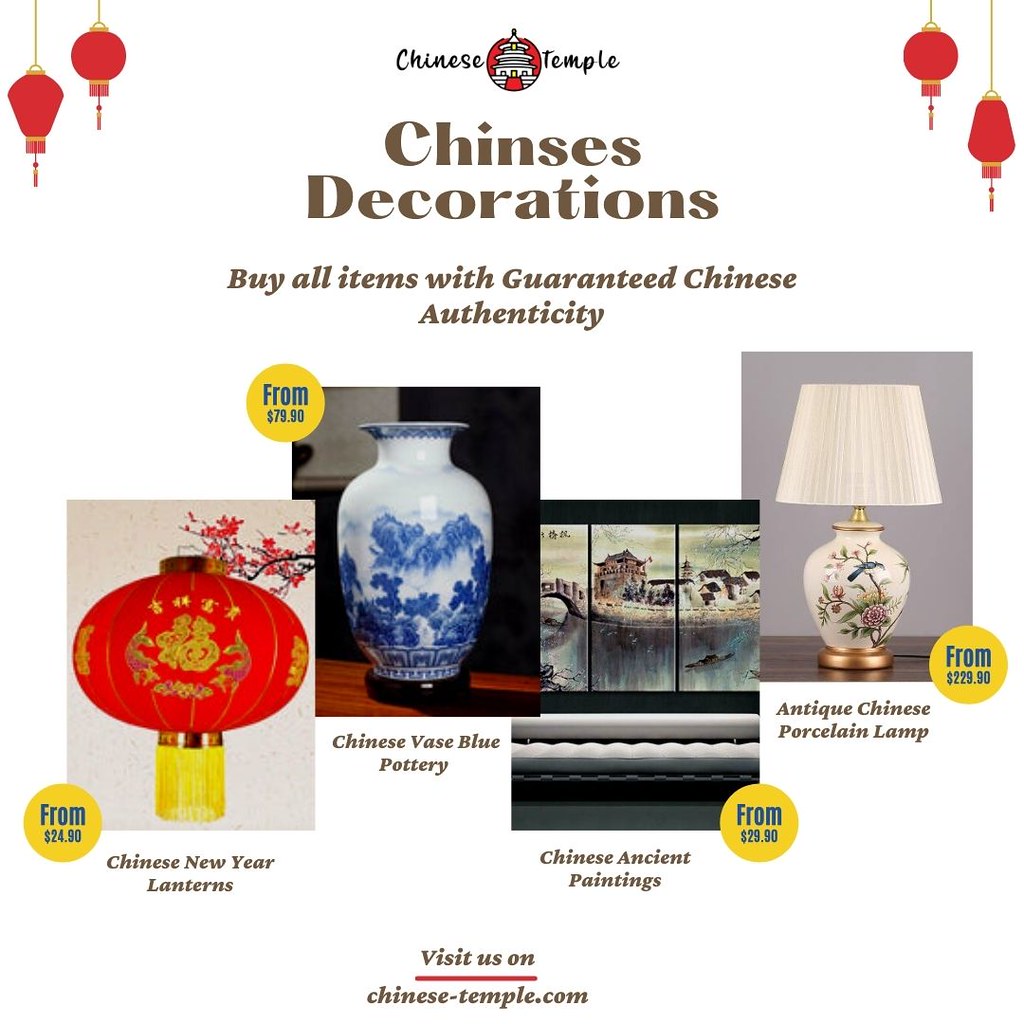The image is an advertisement for various decor items themed around Chinese culture, prominently marketed under the brand "Qin Sees Decorations" (spelled "C-H-I-N-S-E-S"). A striking header reads "Chinese Temple" in a cursive black font, with a circular logo depicting a castle placed between the words "Chinese" and "Temple." This is followed by a tagline in brown font that reads, "buy all items with guaranteed Chinese authenticity."

Central to the advertisement are two lanterns situated in the top left and top right corners; these are stylized as 2D hand-drawn renditions in red with gold borders and strings.

The advertisement showcases four items, each presented with an accompanying photograph, a yellow circle indicating the price, and a brown caption describing the item. 

1. **Chinese New Year Lanterns** - Priced from $24.90.
2. **Blue Chinese Vase** - Priced at $7.90. This vase is a striking piece of blue pottery.
3. **Chinese Ancient Paintings** - Priced from $29.99. The image shows a depiction of water and an Asian, specifically Chinese, building.
4. **Antique Chinese Porcelain Lamp** - Priced at $29.90, featuring a white lampshade adorned with floral patterns.

At the bottom of the image, there is a call to action to visit their website, "Chinese-Temple.com."